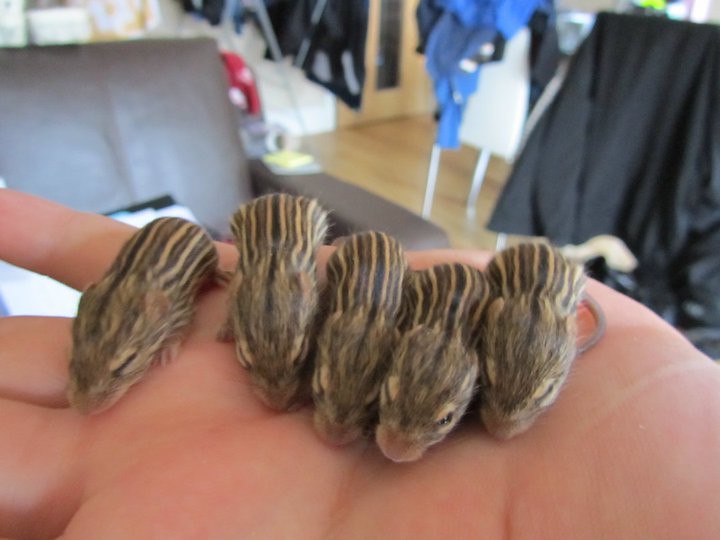This photograph captures an intimate moment where a light-skinned individual cradles five tiny baby animals, likely mice, in their palm. The creatures, each about an inch long, nestle closely together with their small paws tipped with pointed fingers. Their fur is primarily light brown, adorned with striking black and tan stripes running down their backs. Most of the babies have their eyes closed, while one appears to be slightly open, adding a hint of alertness to the group. Their long, thin, pink tails drape delicately over the person's hand. The baby mice have, notably, pink or whitish noses, which they point downward into the palm.

The backdrop presents a cozy, indoor setting, subtly out of focus to emphasize the foreground. On the left, a brown leather chair is partially visible, and on the right, a white chair is laden with a dark blue jacket and another black garment. A wood floor extends beneath a light brown wooden door, which features a small rectangular window. The overall scene, with hints of furniture and clothing, suggests the comfort and warmth of a lived-in space, possibly an apartment.